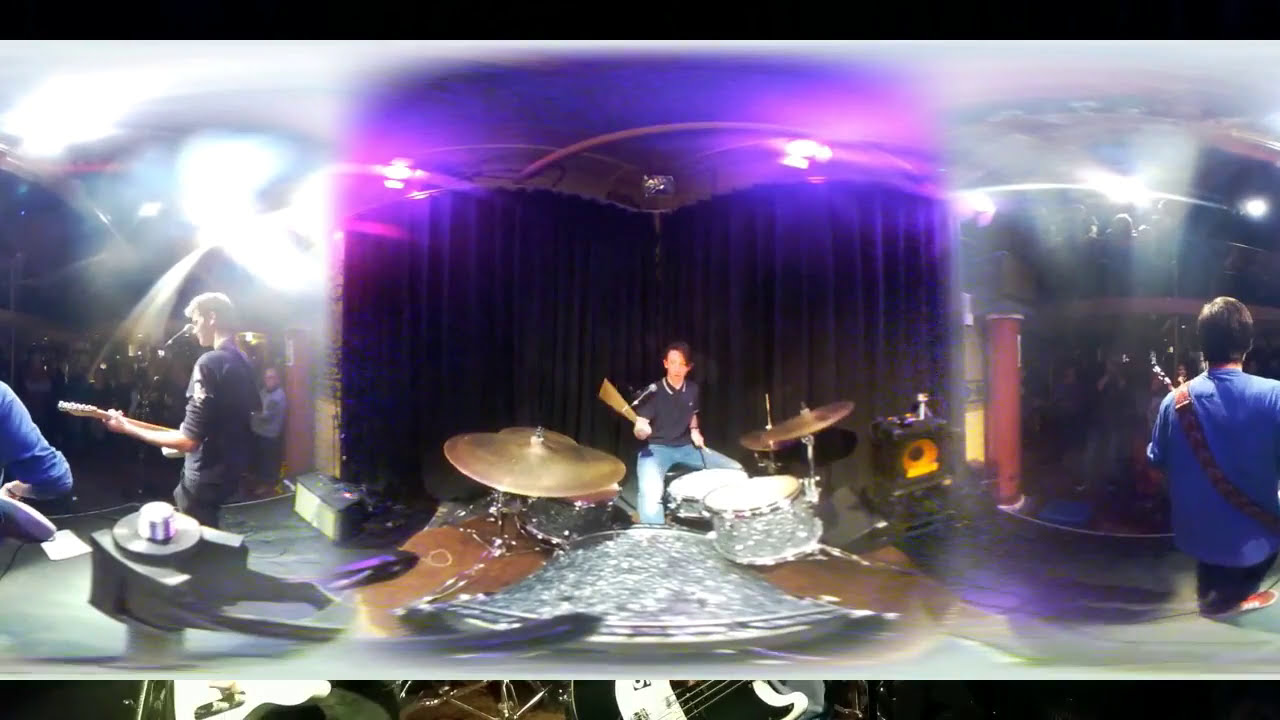This panoramic image captures a dynamic scene of a band performing on stage. At the center, a drummer with dark hair, clad in a black t-shirt and blue jeans, is engrossed in his performance on a silver drum set. The stage is framed by thick blue curtains, and an array of spotlights casts blue and purple hues, creating a vibrant and blurred backdrop. To the right, there's a musician viewed from behind, wearing a blue shirt and dark pants, with a shoulder strap suggestive of a guitar. Beyond him, a small, engaged audience watches the performance. On the left side, you see the edge of the stage where another guitarist, dressed in a dark shirt, plays illuminated by the spotlights. Nearby, a microphone is faintly visible in front of his face, and there are indistinct figures, possibly other performers or equipment, surrounding him. The entire image is bathed in a mix of white, blue, and purple lights from the ceiling, enhancing the lively atmosphere of the event.